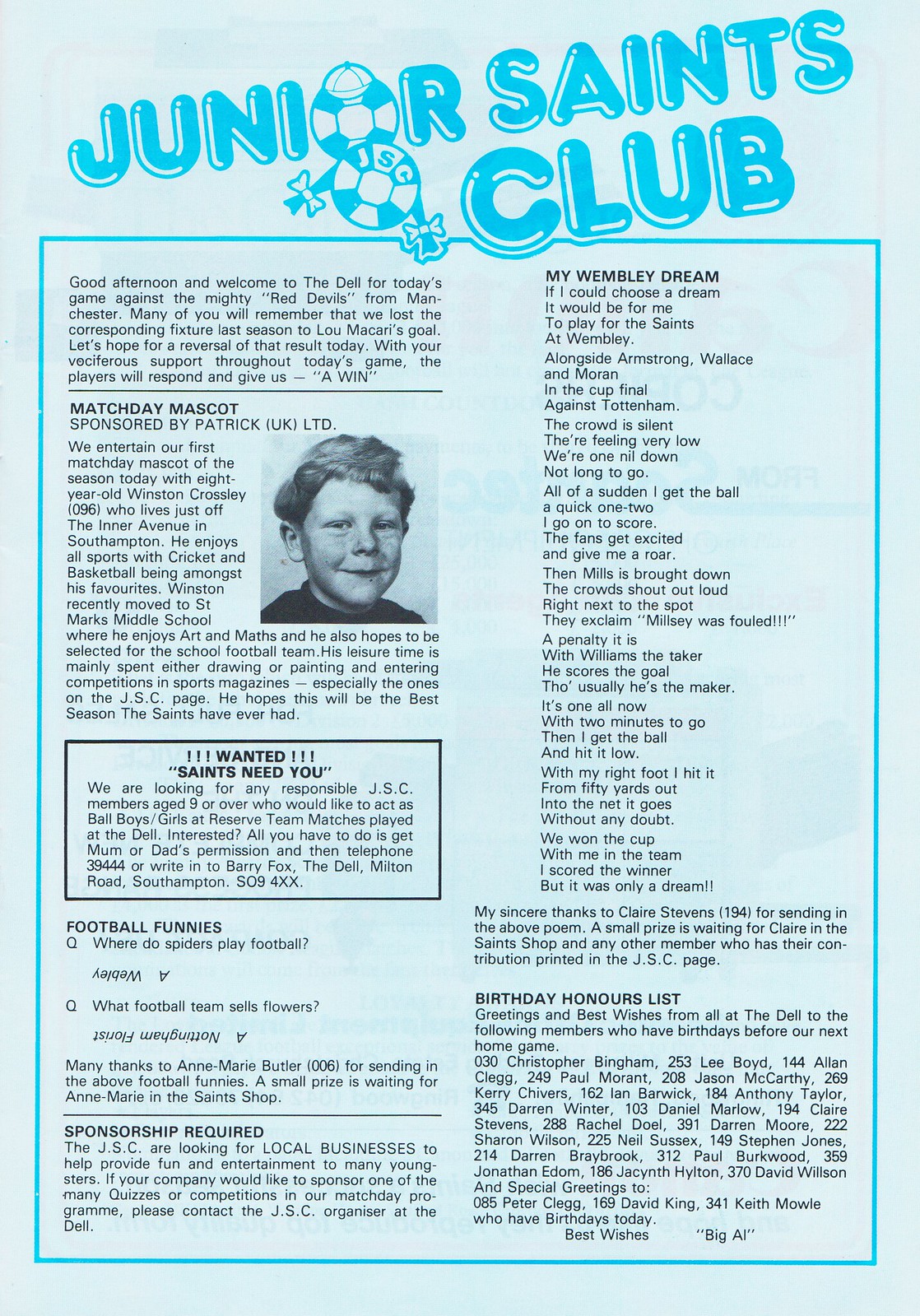The image shows a vertically aligned rectangular flyer with a light blue background, bordered in blue, and takes up the entire frame. At the top, in playful blue bubble letters, it reads "Junior Saints Club" with the 'O' replaced by a soccer ball wearing a baseball hat. Below this heading, the flyer is divided into sections: 

- A paragraph greets the club members and welcomes them to the game against Manchester’s Red Devils, recalling a previous match and rallying for support.
- The "Match Day Mascot" section, sponsored by Patrick UK LTD, features a smiling preteen boy with fluffy brown hair.
- A section titled "Wanted: Saints Need You" followed by a recruiting paragraph.
- Another section named "Football Funnies."
- A line separating it from "Sponsorship Required."

On the right side is a vertical column starting with "My Wembley Dream," introducing several lines of what appears to be a poem. At the bottom, the flyer lists a "Birthday Honors List" with several names. The colors used predominantly include various shades of blue, gray, and black. This flyer seems to be part of a soccer program handed out at a stadium.